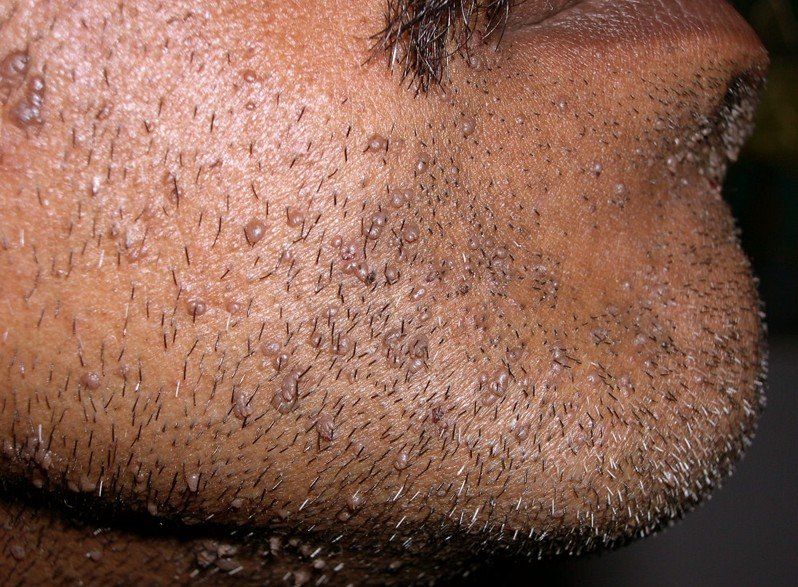The image is a detailed close-up photograph of the side of a man's face, specifically focusing on his chin, which is angled upwards. His skin is a light brown tone and is covered with a mix of short black and gray stubble. The gray hairs are more prominent on the chin, while the cheek, partially visible, has mostly dark hairs. The lower lip, appearing red, is visible in the upper right-hand corner, along with the edges of a mustache composed of longer black hairs. Scattered across the skin are small bumps, resembling very mild acne or possibly a rash, giving the skin a slightly uneven texture. The backdrop of the image is a dark, charcoal color, with the majority of the frame occupied by the man’s skin, leaving minimal background visible. The lighting casts a shadow on the lower part of his neck, which is discernible at the bottom left corner of the image.